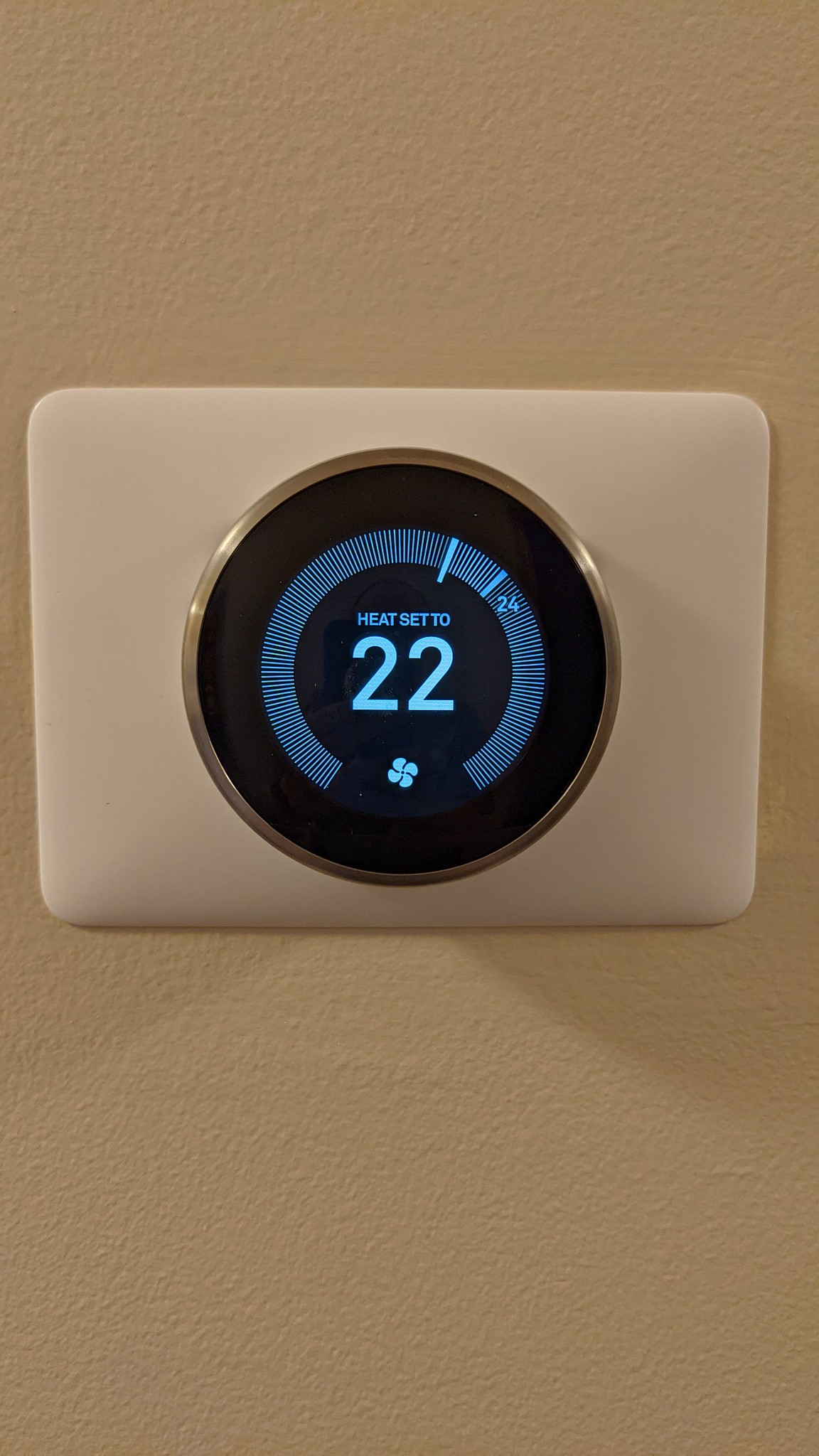This photograph features a sleek electronic thermostat, meticulously mounted on an off-white, textured wall. The thermostat has a rectangular shape and is encased in smooth, white plastic. At its center, a prominent chrome circle, likely made of metal or chromed plastic, serves as the eye-catching focal point. Within this circle is a large, black dial featuring a black background illuminated by light blue text and indicator lines arranged in a circular pattern.

At the bottom of the dial, a small four-bladed fan symbol, rendered in the same light blue color, is clearly visible. In the middle of the dial, the display reads "Heat set to 22," accompanied by a series of blue bars indicating the current temperature setting. The bars align closely with the 22 marker, although some extend further, adding visual complexity to the gradation lines, which do not bear numerical labels. To the right, the number 24 subtly hints at additional settings, contributing to the modern and functional design of the thermostat.